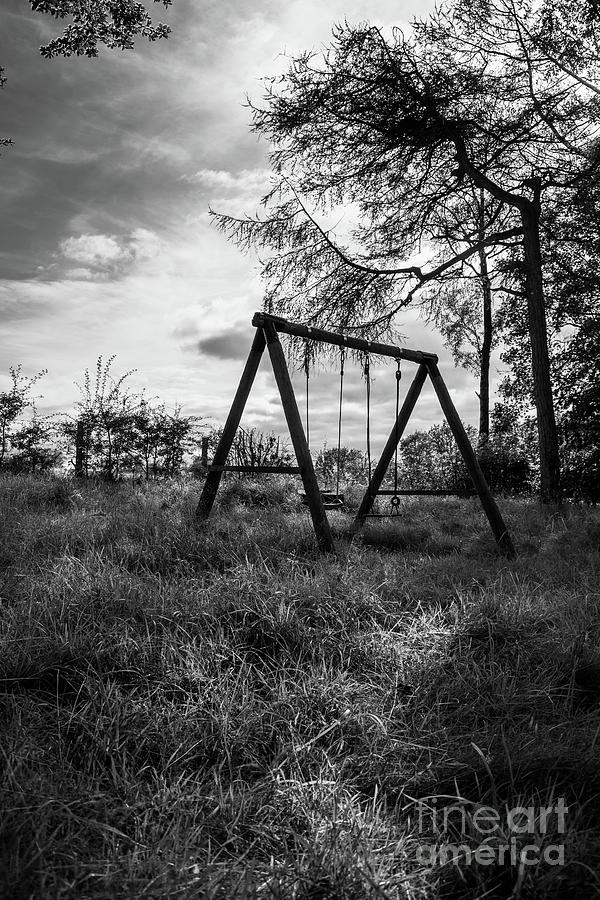In this evocative black and white photograph, a solitary swing set stands amidst an overgrown, grassy field, suggesting abandonment. The swing set, rendered in stark silhouette, features two swings—one appears to be a flat board, the other a bucket seat. Tall, unkept trees form the background, casting long shadows due to the low angle of the sun, indicative of either dawn or dusk. The sky overhead is filled with dark, brooding clouds, enhancing the desolate and melancholy atmosphere. In the lower corner, a Fine Art America watermark is subtly visible, adding to the image’s artistic quality.